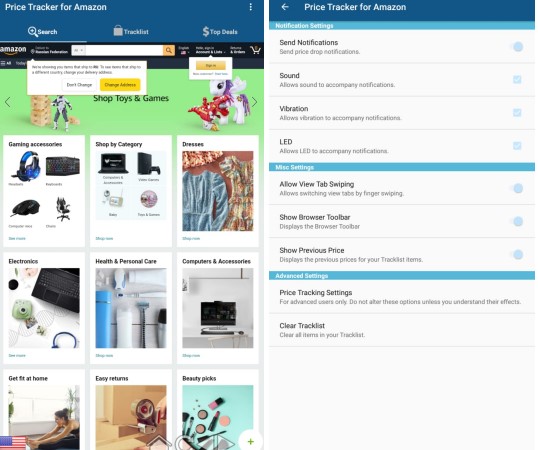**Detailed Caption:**

The image contains two distinct screenshots. 

On the left side, the screenshot features a blue banner at the top labeled "Price Tracker for Amazon". Directly below the banner, there are three tab options: "Search" on the left, "Track List" in the middle, and "Top Deals" on the right. The Amazon website is visible underneath, showcasing its black navigation bar with "Amazon" on the far left, a search bar in the center, and icons for the cart and language settings (American English) on the right. A prompt to change the address appears, stating "Don't change your address." Lower on the page, various product boxes are displayed beneath a green banner promoting "Shop Toys and Games," which includes images of an action figure, a pony, and more. Further down, there are categorized sections such as Gaming Accessories, Shop by Category, Dresses, Electronics, Health and Personal Care, Computers and Accessories, Get Fit at Home, Easy Returns, and Beauty Picks. An American flag is seen in the bottom left corner.

The screenshot on the right side also has a blue banner at the top that reads "Price Tracker for Amazon," accompanied by a leftward-pointing arrow. Below the banner, the interface indicates it is in the "Settings" section with subsections including "Notification Settings," listing various options, "Miscellaneous Settings," with additional options, and "Advanced Settings," which specifically feature "Price Tracking Settings" and "Clear Track List."